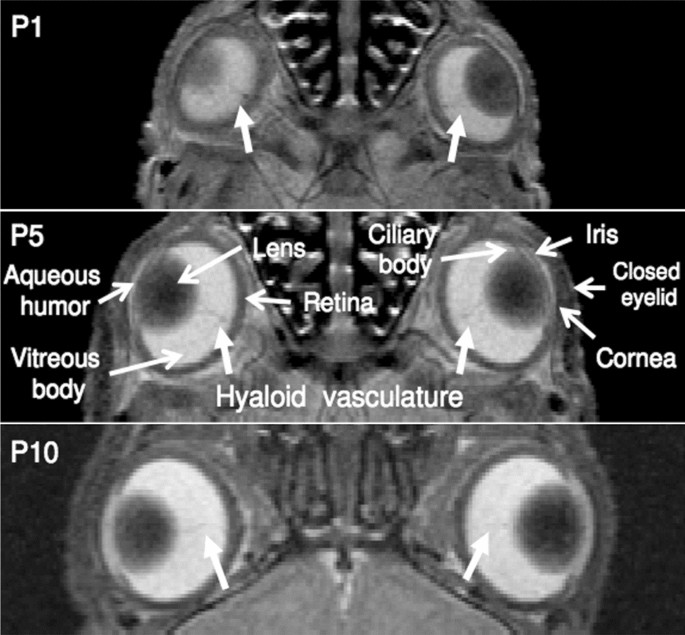The image is a detailed X-ray examination of eyeballs, divided into three horizontal sections. The top section, labeled P1 in the top left corner, displays a standard X-ray where both eyeballs and part of the brain between them are visible. Two arrows point to each eyeball. The middle section, labeled P5, is a zoomed-in version of P1, showing a more detailed X-ray with multiple labeled anatomical features. These include the lens, aqueous humor, vitreous body, hyaloid vasculature, retina, ciliary body, iris, closed eyelid, and cornea, with corresponding arrows pointing to each feature. The bottom section, labeled P10, offers a further zoomed-in view, focusing specifically on the eyeballs with arrows indicating various details. It appears that this is not a human specimen.